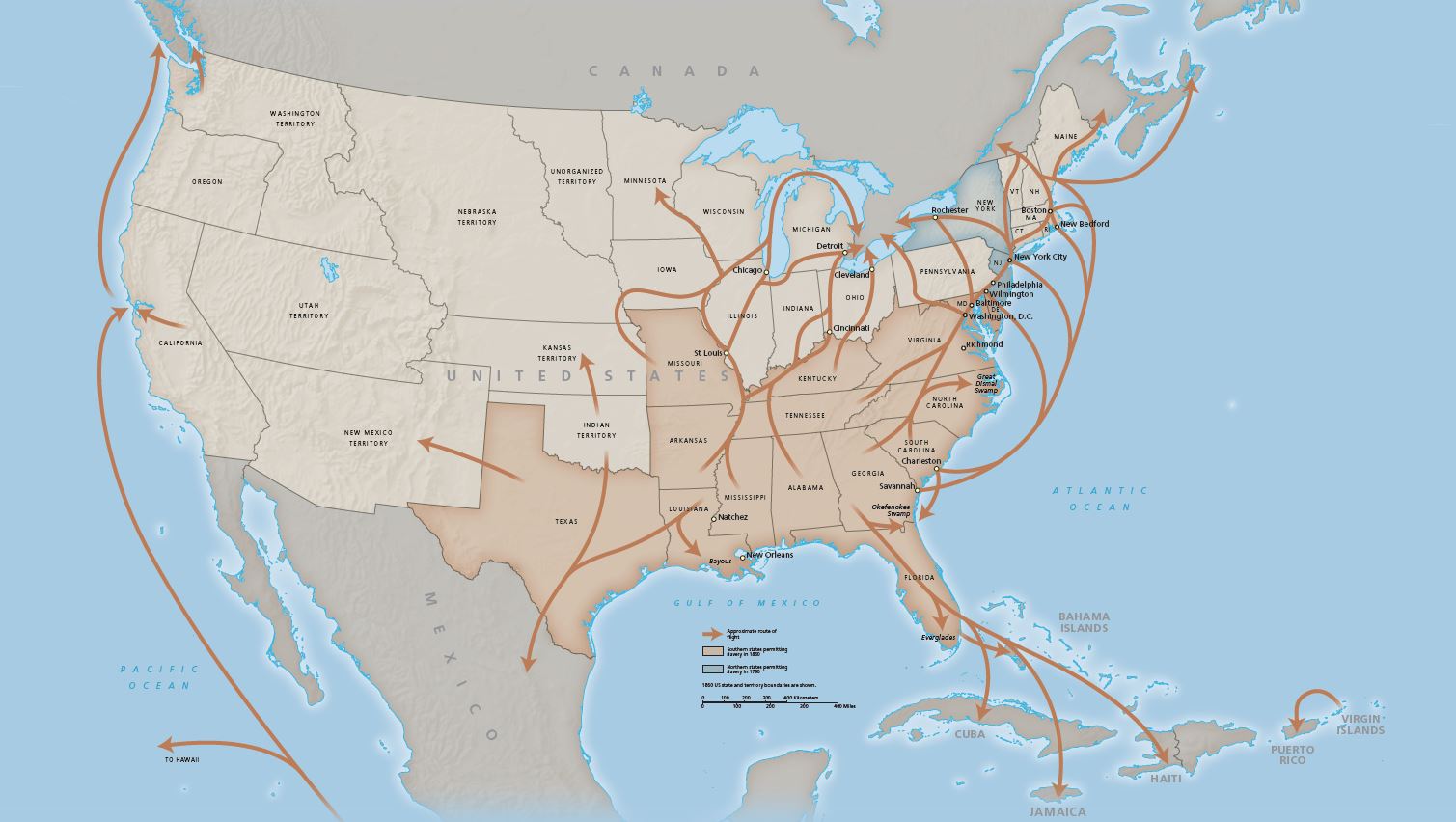This detailed image presents a map of the United States, highlighting several geographical and visual features. The map includes parts of Canada and Mexico, with Canada colored in a grayish tone and Mexico in a similar gray shade. The United States is divided into regions with different colorations: the western states, from Washington State down to California and stretching northeastward, are illustrated in a light beige or khaki brown; the southern states, including Texas, Mississippi, Alabama, Louisiana, Georgia, and the coastal Carolinas, are depicted in a darker beige or tannish brown color. The map meticulously labels each state in black for clarity.

Overlaid on the map are numerous orangey-brown arrows, suggesting patterns that could be indicative of wind, weather fronts, or possibly migration routes. These arrows create a dynamic visual, flowing in varied directions. On the west coast, they trace a path from Mexico to central California, then extend northward to Canada. The Midwest and east coast feature a denser array of arrows, many converging towards the Great Lakes. Arrows also travel from the southern United States, up the eastern seaboard, with several pointing towards different northeastern states and extending to Canada. Additionally, some arrows move from Florida southwards to the Caribbean, including Cuba, Jamaica, and Haiti, visible in the bottom right corner beside the Atlantic Ocean. The surrounding waters, presumably the Atlantic Ocean, frame the detailed and meticulously designed map.